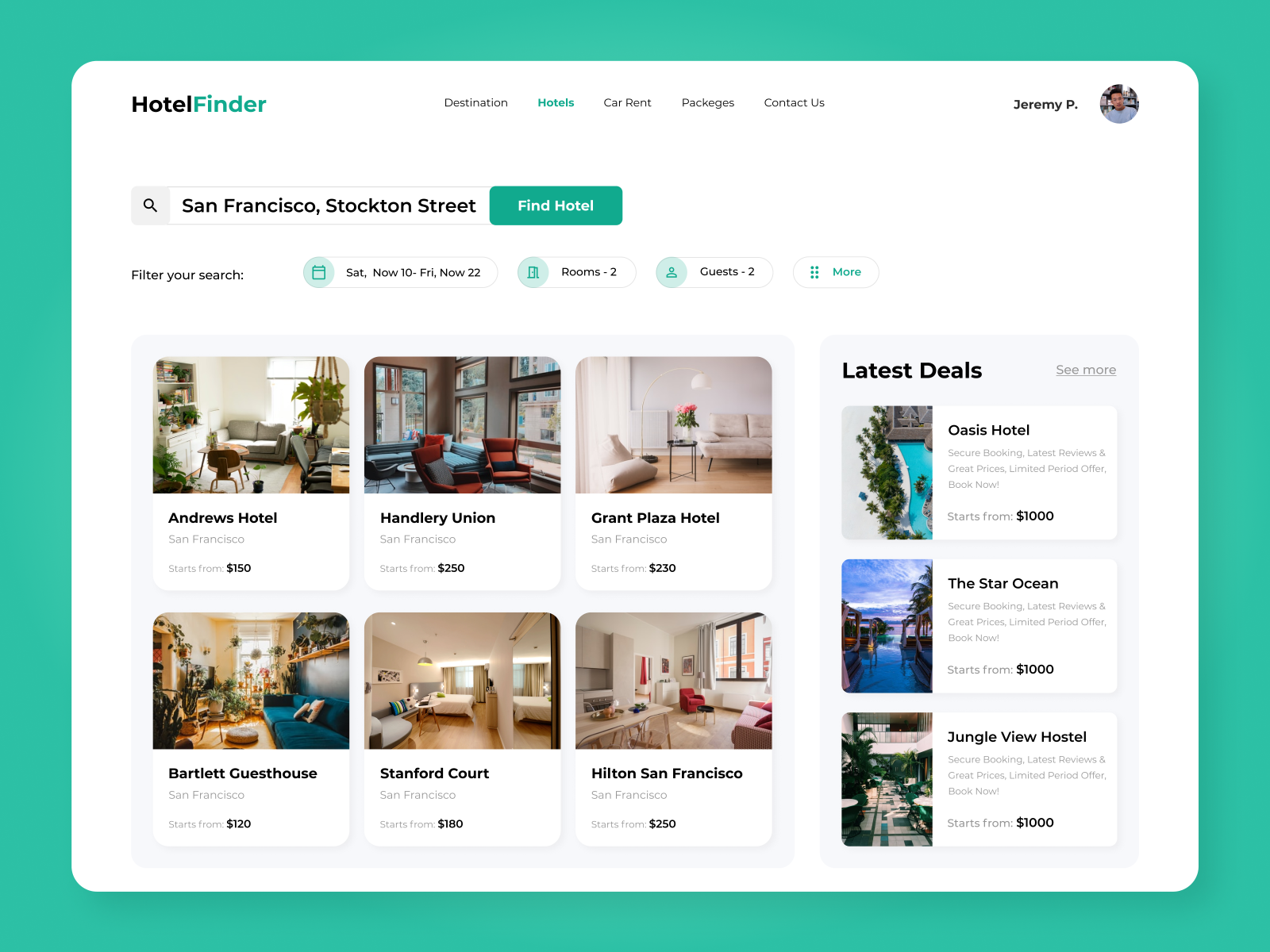The image depicts a web page designed as a hotel finder platform. The page features a prominent square bordered by a thick mint green line, enclosing a white information box. In the top left corner of this box, the header "Hotel Finder" is displayed. Below this, navigation options are sequentially listed: "Destination," "Hotels," "Car Rent," "Packages," and "Contact Us." Further down, a white space precedes the display of "Jeremy P." accompanied by his profile picture.

The main interactive element on the page is a search box where users can input their desired hotel location. Underneath, several search filters are provided, allowing users to specify dates, number of rooms, and number of guests. An additional dropdown menu is available for further filtering options.

Displayed below these filters are two rows of hotel options, with three hotels per row, totaling six featured hotels: Andrews Hotel, Handlery Union, Grant Plaza Hotel, Bartlett Guesthouse, Stanford Court, and Hilton San Francisco. There is also a section labeled "Latest Deals," presenting three special offers on hotels (not shown in the image). A clickable shaded vertical rectangle labeled "See More" invites users to explore additional deals.